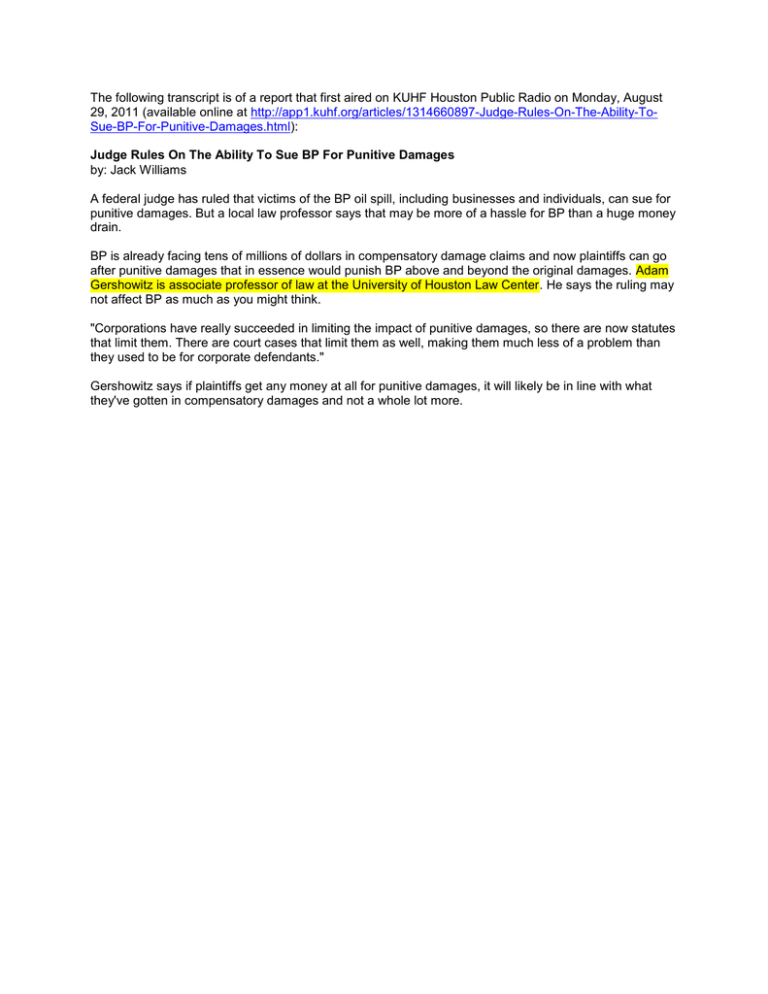Starting from the top area with black text, the image captures a transcript from a report that aired on KUHF, Houston Public Radio, on Monday, August 29, 2011. The text is also available online at KAHF Organized Articles under the title "Judge Rules on the Ability to Sue BP for Punitive Damages," authored by Jack Williams. The report details that a federal judge has ruled that victims of the BP oil spill, including businesses and individuals, are entitled to sue for punitive damages. However, Adam Gochowicz, an Associate Professor of Law at the University of Houston Law Center, comments that this ruling may be more of an administrative hassle for BP rather than a substantial financial threat. Despite the new ability to pursue punitive damages aimed at punishing BP beyond the original claims, corporations, including BP, have been effective in minimizing the impact of such penalties through existing statutes and court cases. Gochowicz emphasizes that these legal limitations have made punitive damages a less significant issue for corporate defendants than they used to be.

The caption could be further illustrated with a highlighted excerpt focusing on Gochowicz’s explanation, shown prominently in yellow text: "Corporations have highly succeeded in limiting the impact of punitive damages, so there are now statutes and court cases that limit them, making them much less of a problem than they used to be for corporate defendants."